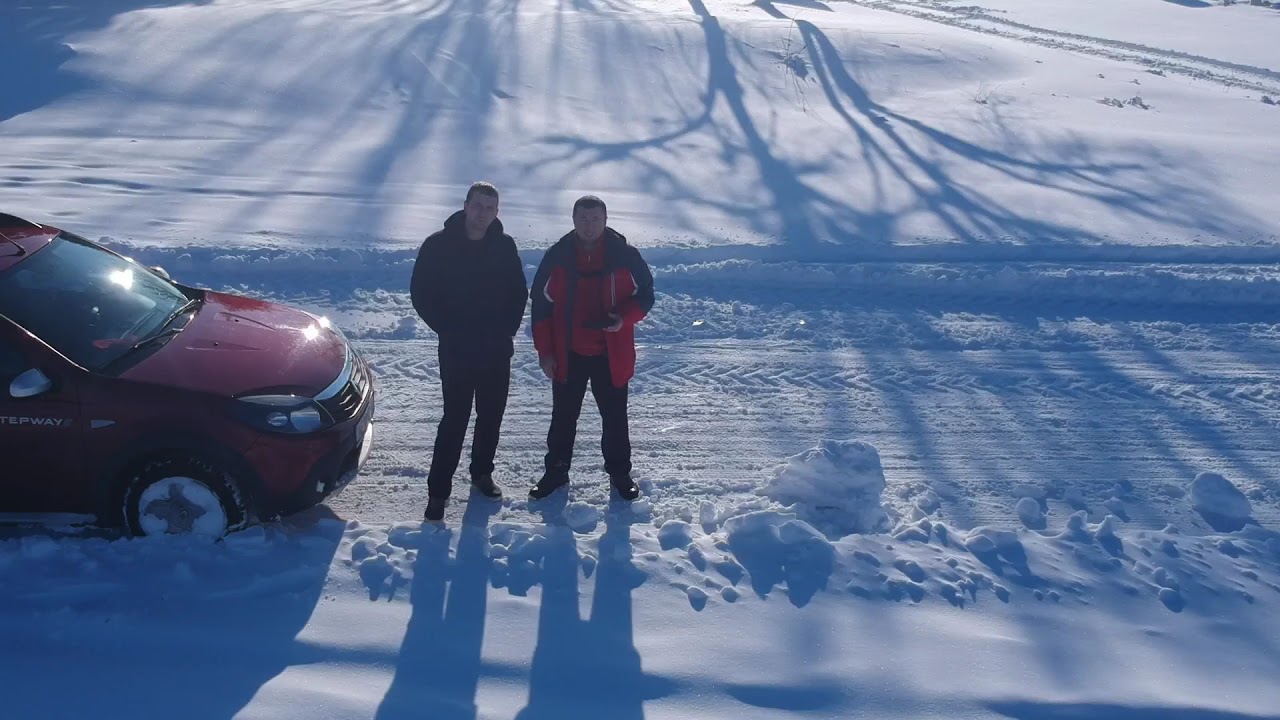This photograph captures a snowy outdoor setting featuring two men standing in the middle of a road blanketed with a thick layer of snow. Both men are facing the camera; the man on the left is dressed in a black coat and jeans, while the man on the right wears a red coat with black pants. The road appears entirely snow-covered, with visible tire marks weaving through the snow, suggestive of recent vehicular movement. To the left of the men is a dark red SUV, its hubcaps and wheel wells bogged down with snow. The bright sunlight casts pronounced shadows of the men and nearby trees that are out of the frame, emphasizing the clear and sunny winter day. Beside one of the men, there are large clumps of hard snow, indicating the cold temperature. One man appears to be holding an indistinguishable object, possibly a controller or camera. The vantage point is such that the sky and any surrounding buildings are not visible, directing full attention to the men, the car, and the snowy expanse.